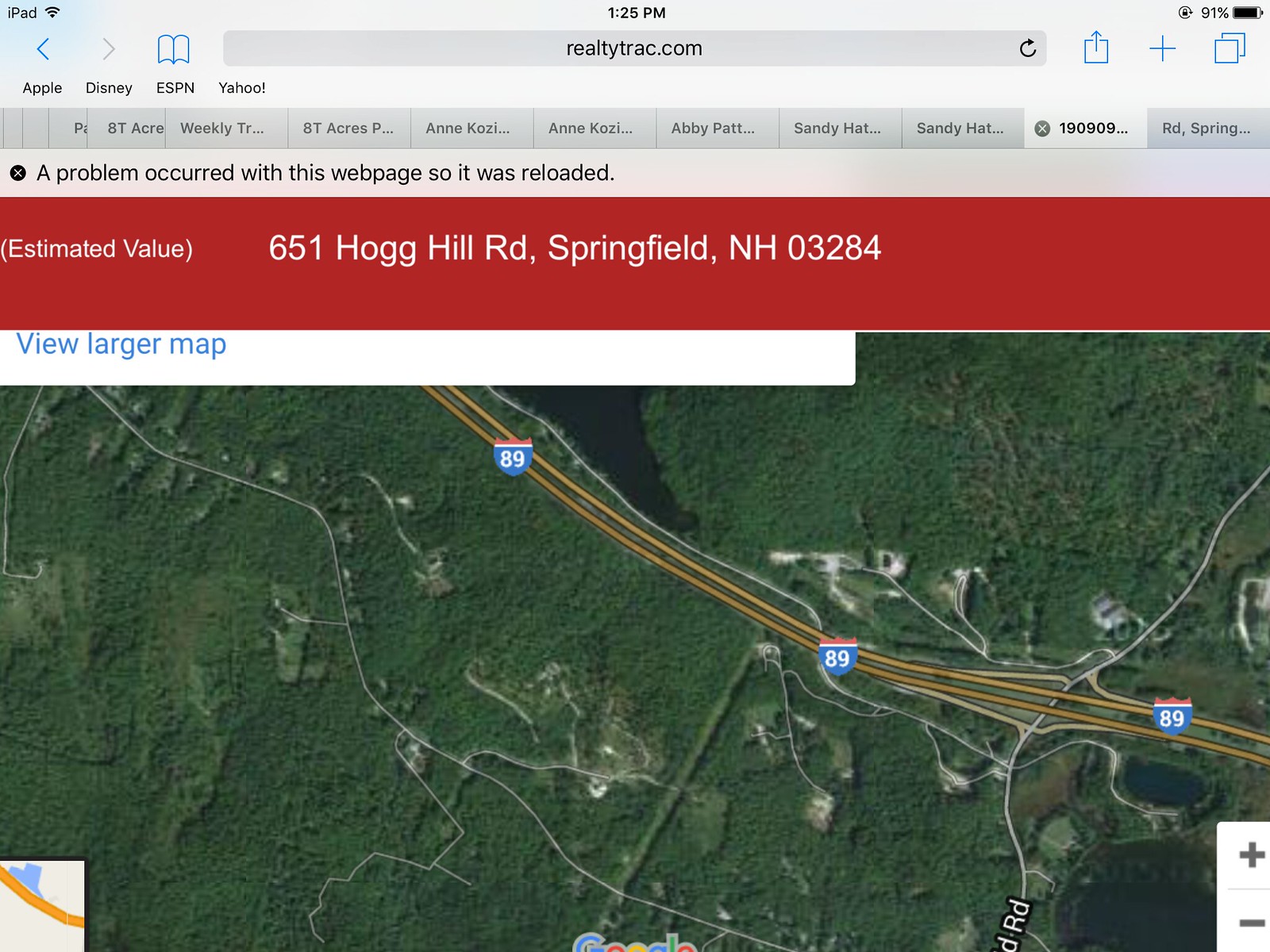This detailed color screenshot captures a landscape-oriented image from an iPad's Safari browser at 1:25 p.m., displaying 91% battery life. The URL bar at the top reveals the website RealtyTrack.com. The page has experienced an issue and was reloaded, indicated by a message stating, "A problem occurred with this webpage, so it was reloaded." Below this message, a bold red strip with white text shows the estimated value of a property located at 651 Hog Hill Road, Springfield, NH 03284. 

Visible underneath is a high-resolution aerial view focusing on the region near Highway 89, which traverses from the top left to the bottom right of the image. The landscape is dominated by dense forests interspersed with two or three small lakes. Additionally, the bottom left corner of the screenshot features a clickable inset map, while the bottom right corner includes zoom in and out buttons represented by a plus and minus sign. The navigational elements on the screen include Apple's first-party apps like Apple, Disney, ESPN, and Yahoo, visible in multiple open windows beneath the main navigation bar.